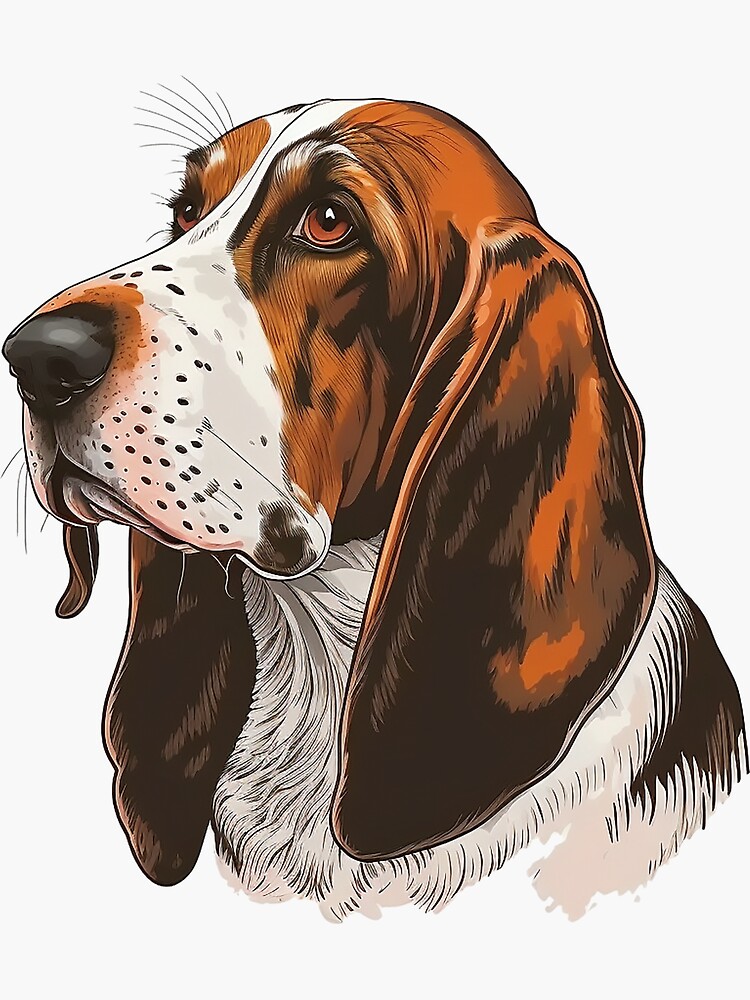This image is an artistic sketch of a beagle, set against a pristine white background. The beagle's head and neck are meticulously detailed while the rest of its body is faded out, leaving a focus on its striking facial features and expressive eyes. The dog has droopy ears and a distinguished side profile facing left and looking upwards. The beagle is primarily brown on its ears, side of the head, around its eyes, and part of its nose. A prominent white stripe runs between its eyes down to its muzzle, which also shows a speckling of small black dots or whiskers. Its chin and neck are white, complementing the white on its chest. The dog's eyes are a bright brown, giving it a lifelike and attentive expression. The overall composition emphasizes the fine details and color contrasts of the beagle's face, making it a captivating piece of art.